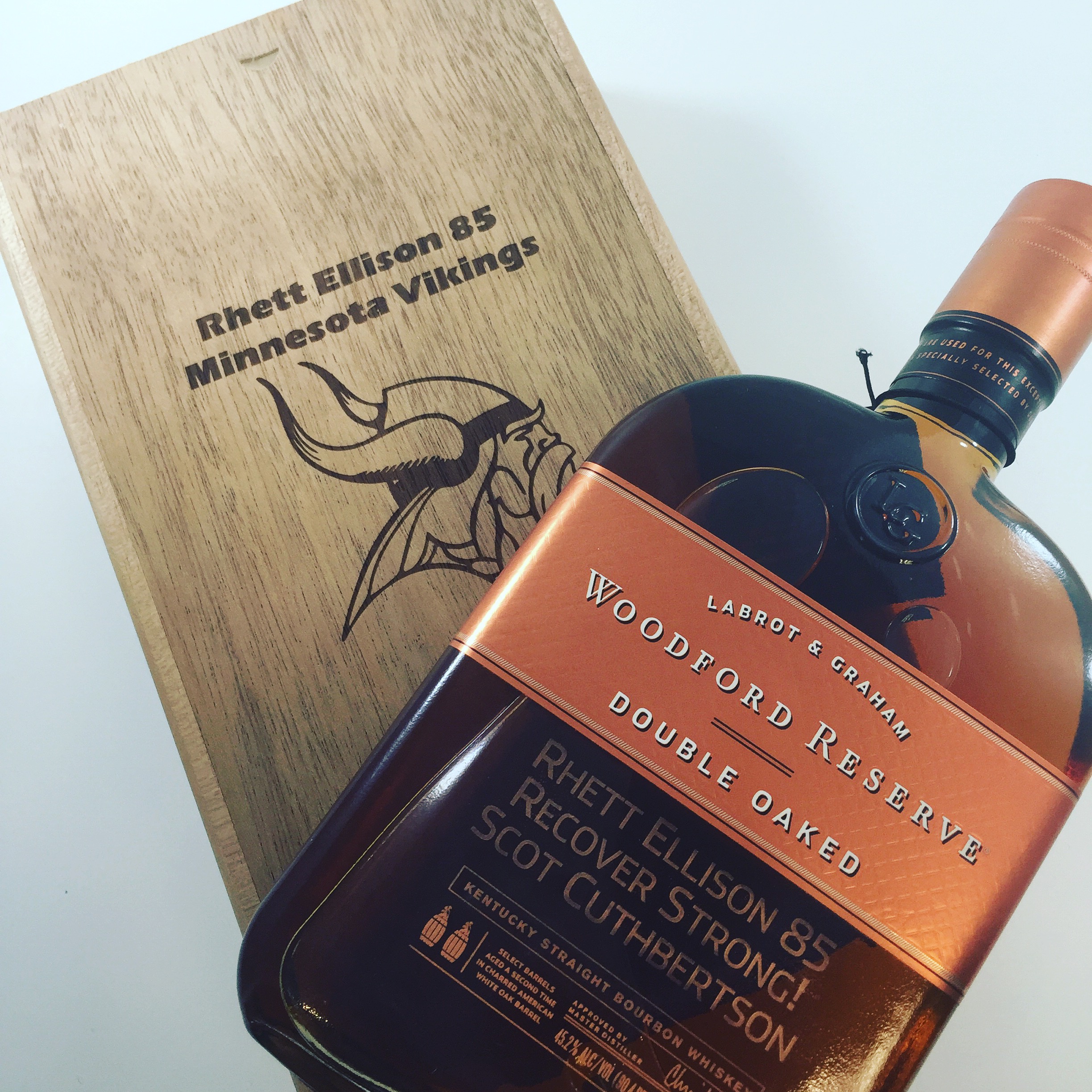In this image, we see a detailed setup featuring a prominent brown liquor bottle positioned towards the bottom right. The bottle is equipped with a maroon-gold band sealing its copper screw-on cap. It bears a detailed label that includes the phrases "Labyrinth and Graham," "Woodford Reserve," and "Double Oaked." The middle section of the label includes additional text, though partially obscured, mentioning "officially selected by" and "Recover Strong" alongside "Rhett Ellison 85."

Behind the bottle, angled towards the top left, is a cutting board or flyer that is light blue in color. Centrally located on this board is the name "Rhett Ellison 85," coupled with references to the "Minnesota Vikings." A detailed illustration of a Viking head, complete with a helmet, horns, and a beard, is prominently featured, facing right. The cutting board serves as both a background and a thematic anchor, connecting the elements of the bottle and the imagery of the Viking together.